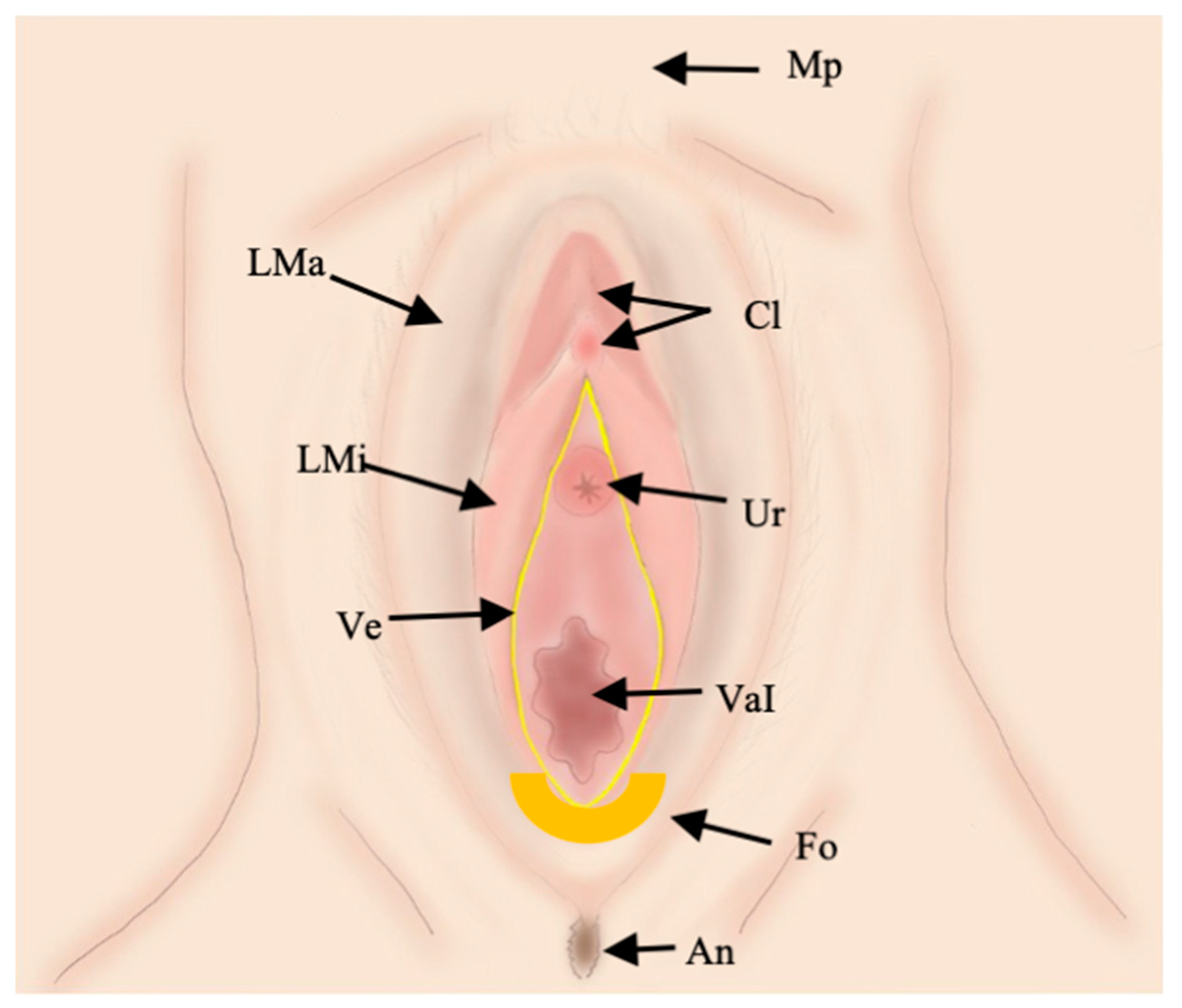The image is a detailed, animated graphic of the female genital area, depicted in a fleshy pink color. It features several black-labeled abbreviations with arrows pointing to specific parts of the anatomy, including MP, LMA, LMI, VE, CLUR, VAL, FO, and AN. The innermost part of the vulva is highlighted with a yellow line, and a yellow half-circle is situated at the bottom of this highlighted region. The visual appears educational, possibly intended for use by medical or anatomy students, and includes light representations of pubic hair. The emphasis on labeling suggests it might be part of a learning exercise or quiz.